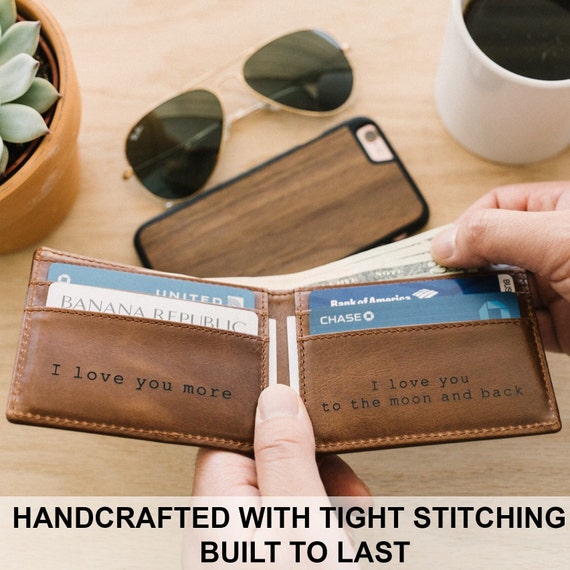The image is a detailed advertisement for a brown leather wallet with a focus on its craftsmanship and sentimental text engravings. The backdrop is a rustic wooden table adorned with several objects, creating a cozy and everyday ambiance. In the top left-hand corner, there is a partially visible potted plant with green leaves in a brown pot. Central to the image are dark aviator sunglasses with metal frames and a cell phone, distinguished by its wood grain case and black rim. In the top right-hand corner, a white coffee mug filled with black coffee is situated. Central to the scene is a man's left hand holding the open wallet, with his right hand pulling out several $20 bills, just the tips of which are fanned out. The wallet, beautifully crafted from brown leather and featuring light brown stitching, displays sentimental black text on the interior: "I love you more" on the left, and "I love you to the moon and back" on the right. Several credit cards are neatly tucked into the wallet's slots, including a green United card, a white Banana Republic card with green font, a green Chase card, and a green or blue Bank of America card. At the bottom of the image, in black font on a white section, the text reads: "Handcrafted with tight stitching, built to last," emphasizing the wallet's quality and durability.